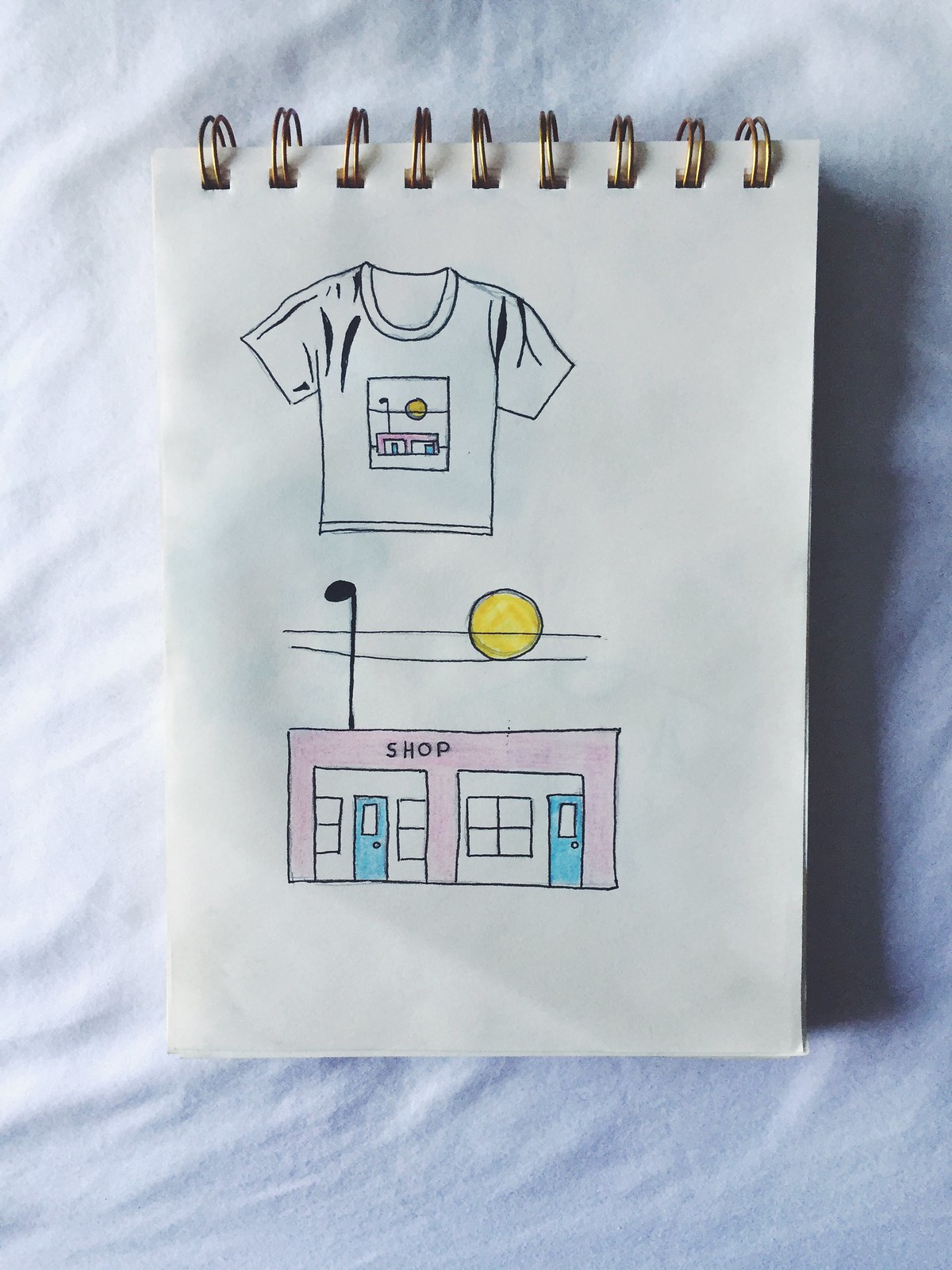A small, rectangular, spiral-bound white notebook rests on a smooth yet slightly wrinkled white fabric, likely a bed sheet. The notebook casts a subtle shadow to its right, accentuating the ambient softness. The notebook's spine is adorned with approximately eight or nine golden double spirals, threaded meticulously through square-shaped holes.

Inside the notebook, an artist's sketch captures the viewer's attention. It depicts a white t-shirt featuring a design that is also replicated below it. The design showcases a charming pink rectangular shop with the word "shop" emblazoned on it. Behind the shop, a black streetlight rises, with two telephone wires stretching across the scene under a bright yellow sun. The shop's façade includes two blue doors, framed by sections resembling white garage doors, which contain additional windows, completing the quaint and colorful storefront illustration.